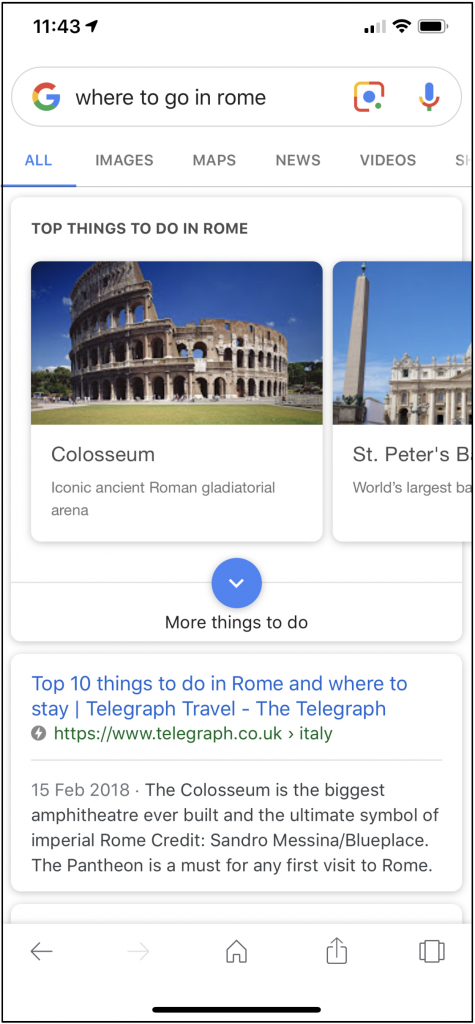The screenshot depicts a website interface framed by a thin black line. At the top of the screen, the time is displayed as "11:43" in black text against a white background. To the right, icons for Wi-Fi signal, cellular signal, and battery status are visible. Below this section, a search bar featuring the Google logo (G) is prominently displayed with the query "Where to go in Rome" entered. A microphone icon is positioned to the right of the search bar. 

Directly below the search bar, navigation options labeled "All," "Images," "Maps," "News," "Videos," etc., are listed, although some are cut off. "All" is highlighted with a blue underline. 

The main content begins with a header titled "Top Things to Do in Rome," followed by listed attractions. The first attraction is "The Colosseum," described as an "iconic ancient Roman gladiatorial arena," accompanied by an image of the Colosseum. Following this is "St. Peter's," though only partially visible, with the description starting as "world's largest" and ending prematurely. 

A blue circle with a downward arrow and the text "More things to do" appears centrally. Below this, a small square section advertises an article titled "Top 10 Things to Do in Rome and Where to Stay." 

A line separates this section from the text "Telegraph Travel - The Telegraph," followed by a link related to the Colosseum. At the bottom of the screen, navigation icons include a left arrow, a house, an upload symbol, and a rectangle with two smaller squares on either side.